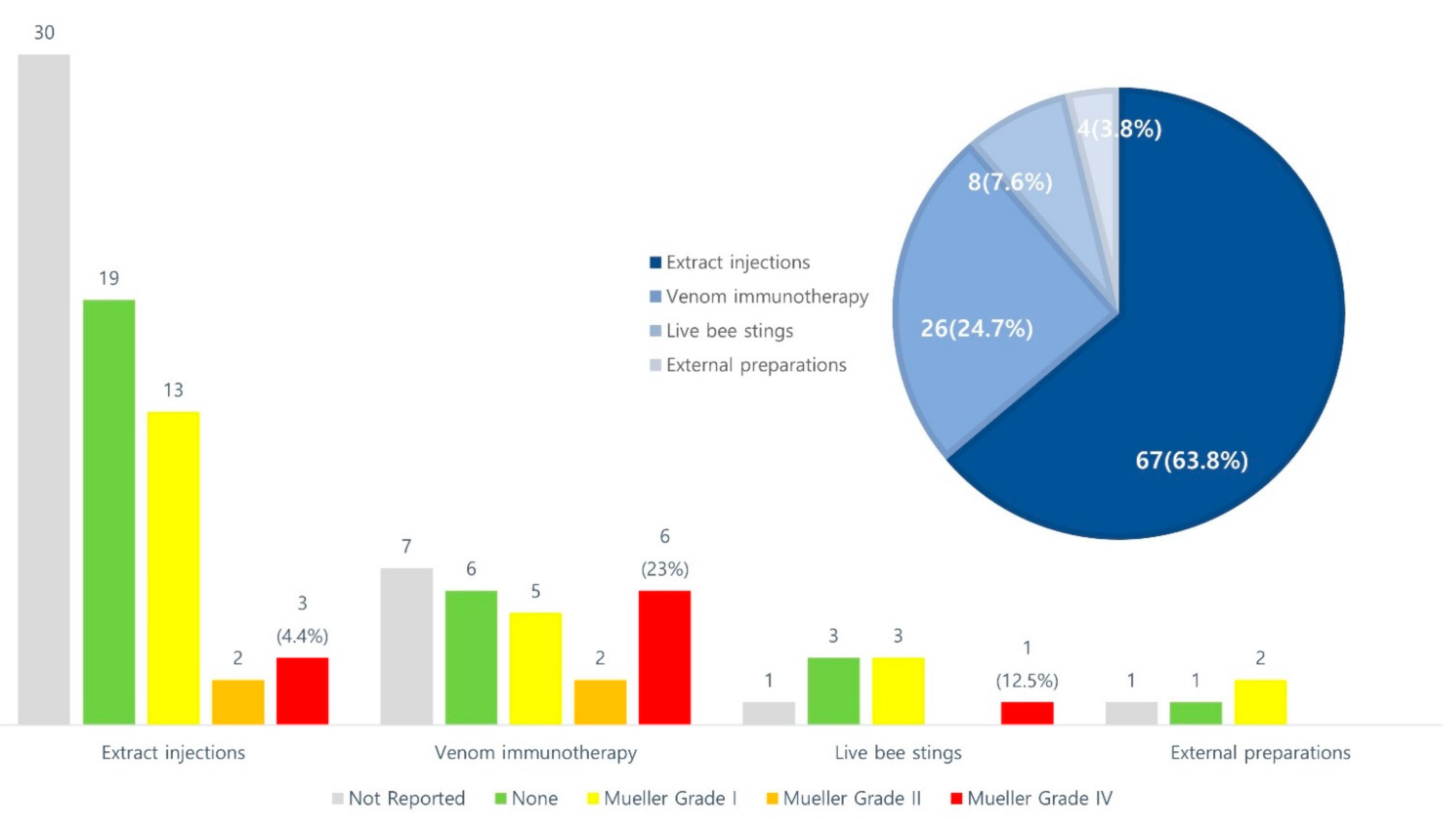This image is an infographic featuring a detailed bar chart and a pie chart, focusing on medical data related to various treatments. The bar chart, displayed in colors of gray, green, yellow, orange, and red, presents data on extract injections, venom immunotherapy, live bee stings, and external preparations. The color-coded categories denote different Mueller grades, with gray indicating 'not reported', green as 'none', yellow as 'Mueller grade I', orange as 'Mueller grade II', and red as 'Mueller grade IV'.

Positioned in the top right corner, the pie chart summarizes the proportional data in shades of blue, transitioning from dark blue to almost a grayish-blue. The largest section of the pie chart, 63.8%, represents extract injections. Venom immunotherapy constitutes 24.7% in a medium blue shade, followed by live bee stings at 7.6% in a lighter blue, and external preparations at 3.8% in a very light blue. The organized layout provides a clear representation and comparison of treatment modalities and their associated data.